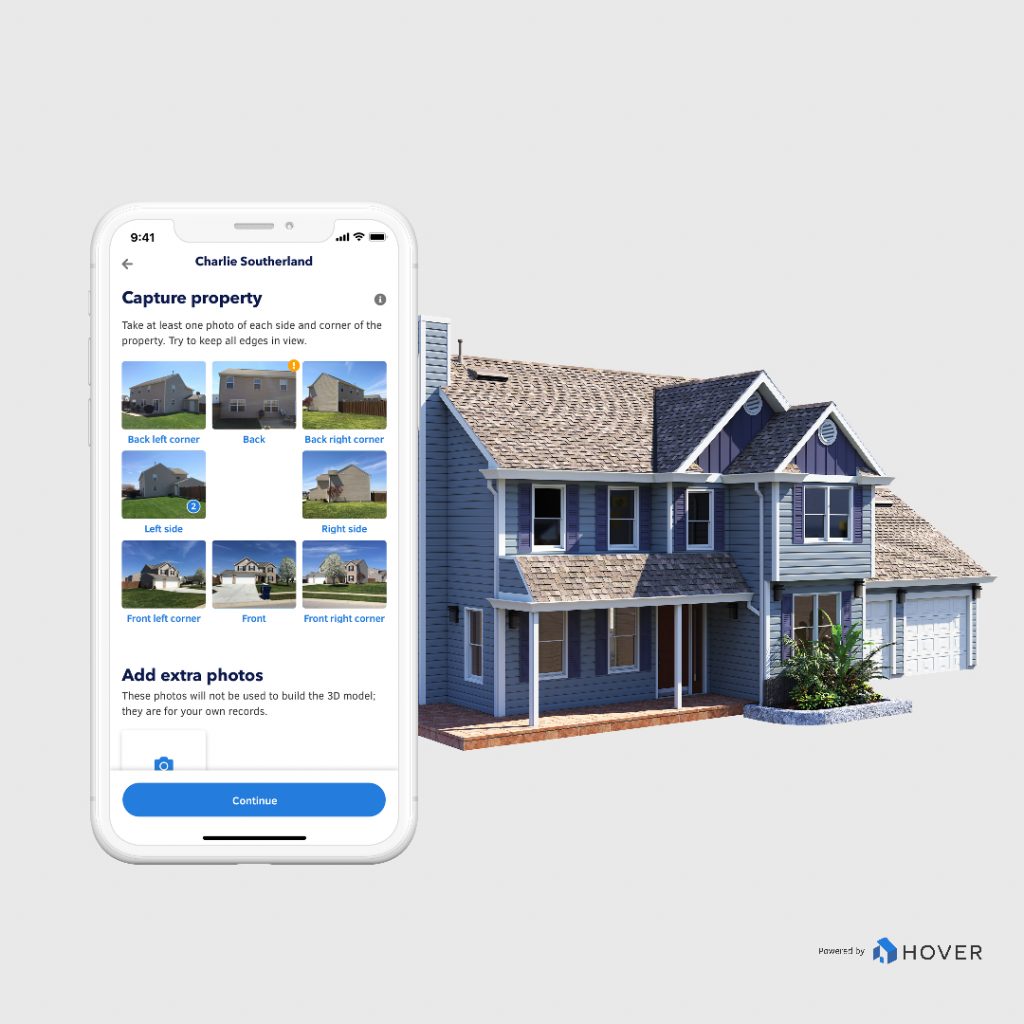The image features a picturesque home with distinctive architectural elements. The house boasts a gray roof, complete with triangle-shaped gables near the front. The exterior is clad in blue siding, complemented by matching blue shutters. A welcoming small front porch with white posts and a two-car garage adorned with white doors add to the charm of the property. To the left of the structure, a chimney discretely rises beside the roofline. A large, verdant plant is positioned in front of a window situated to the right of the front door, enhancing the home's curb appeal.

Additionally, the image includes a snapshot of a cell phone displaying instructions from Charlie Sutherland about capturing property images. The guidelines emphasize taking photos from various angles, including the back, back right center, left side, right side, front, front left corner, and front right corner. These images should clearly display all edges of the property. It also suggests adding extra photos for personal records, noting that these will not be used to construct the 3D model. At the bottom right corner of the cell phone screen, the "Hover" program is mentioned, with a blue 3D shape icon beside the word "Hover."